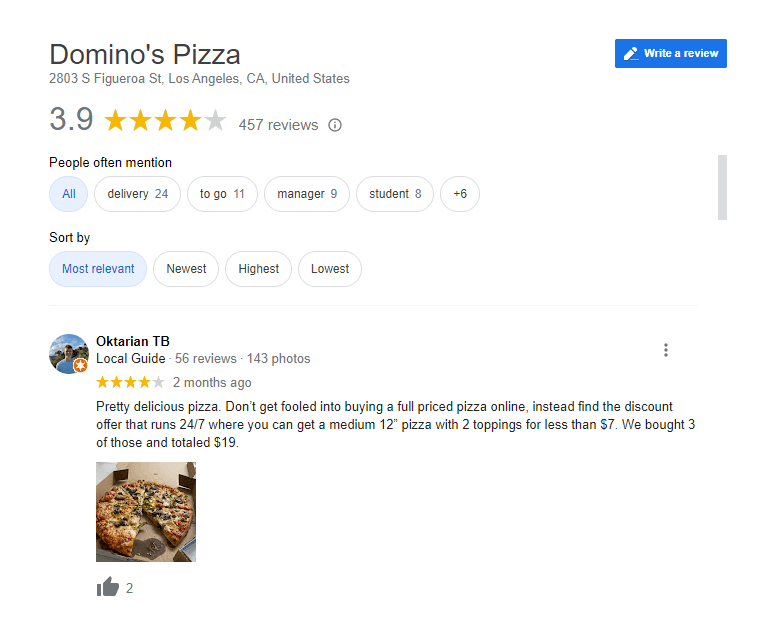This image showcases an online advertisement and review summary for Domino's Pizza, specifically for the location at 2803 South Figueroa Street, Los Angeles, California, USA. 

**Left Panel:**
- The heading displays "Domino's Pizza" in black text.
- Below the heading, the address "2803 South Figueroa Street, Los Angeles, California, United States" is listed.
- Further down, a rating of 3.9 out of 5 stars is highlighted, based on 457 reviews.
- The section titled "People Often Mention" features frequently discussed keywords with their mention counts:
  - Delivery: 24 mentions
  - To Go: 11 mentions
  - Manager: 9 mentions
  - Student: 8 mentions
  - There are six more unspecified mentions, with "All" chosen as the selected filter.

**Right Panel:**
- A blue box with white text urges users to "Write a Review."

**Bottom Section:**
- A featured review by Octarian TV, a Local Guide with 56 reviews and 143 video photos.
- The review, rated 4 stars out of 5 and posted two months ago, reads: "Pretty delicious pizza. Don’t get fooled into buying a full-price pizza online. Instead, find the discount offer that runs 24-7 where you can get a medium 12-inch pizza with two toppings for less than $7. We bought three of those and totaled $19."

Additionally, options exist to sort reviews by "Most Relevant," "Newest," "Highest," and "Lowest."